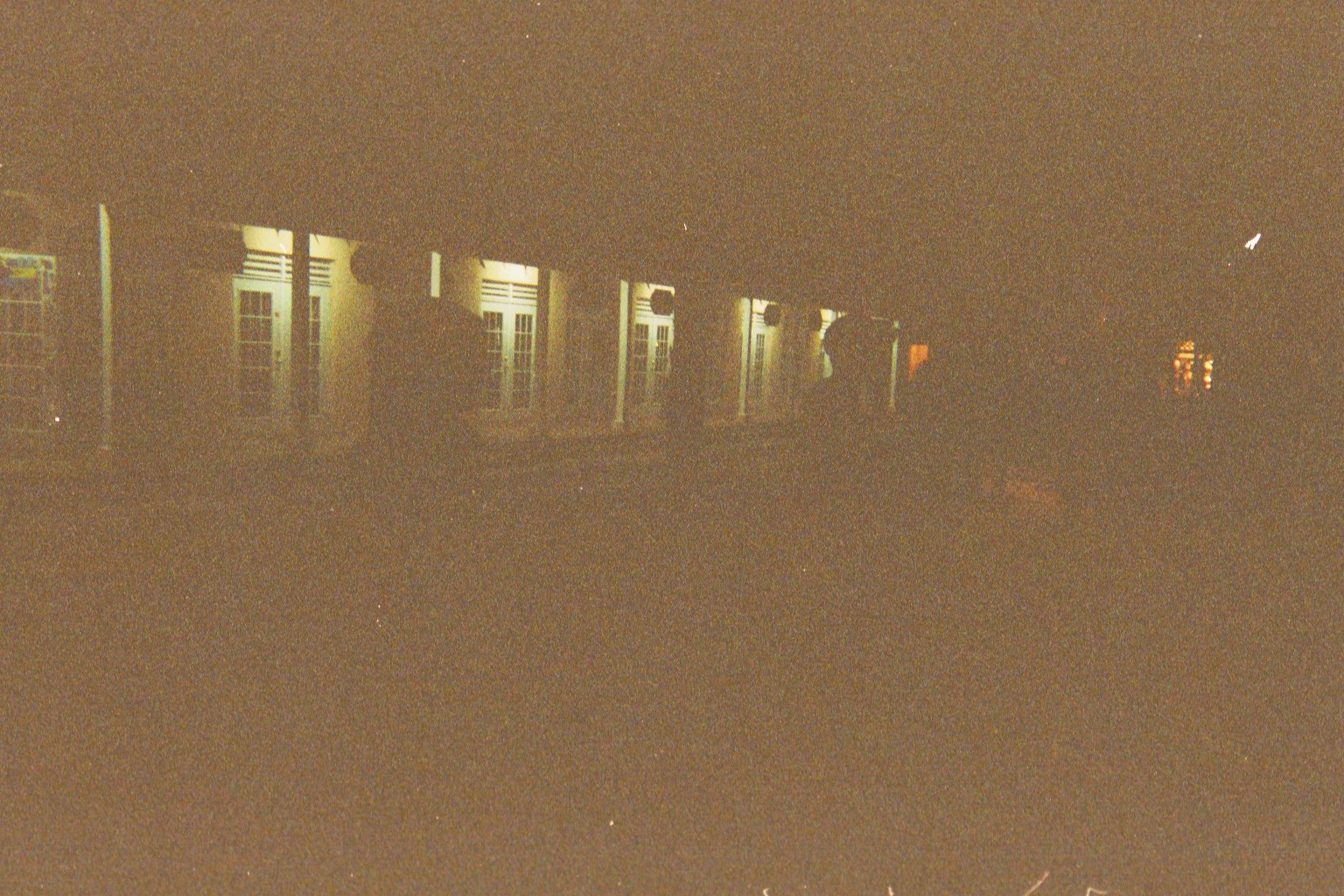This color snapshot photograph, likely taken with a high-speed film resulting in an incredibly grainy texture with dot patterns throughout, depicts the dimly-lit exterior of a building at night. The setting resembles the bottom tier of a building, possibly an apartment complex or a banquet hall, featuring multiple glass-panelled double doors – specifically, five pairs are clearly visible with an additional one receding into the distance. Each doorway is illuminated by a small spotlight mounted above it. On the far right, faint orange lights possibly from nearby houses are noticeable. The scene includes a couple of shadowy figures walking in the foreground, their silhouettes partially identifiable against the door lights. Additionally, a vending machine can be seen on the left side of the building. The overall darkness and silhouetted forms give the impression of an incompletely developed film photo, contributing to the image's blurry, saturated, and somewhat eerie aesthetic.